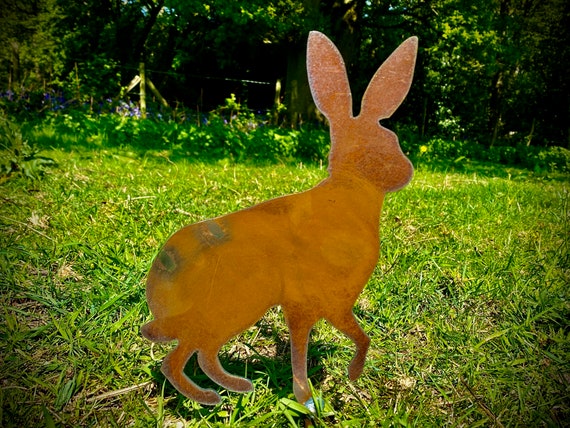The image captures a picturesque, grassy backyard typical of a rural setting. The foreground showcases an intricately detailed metal cut-out of a bunny rabbit, centered with its ears perked up and facing right. Despite some wear and signs of rust, the silhouette remains distinct with three paws on the ground and one raised, lacking facial features and texture. Surrounding this central figure, the yard is lush with green grass interspersed with brown patches. The upper portion of the image transitions into a densely treed area, punctuated with purple flowers that stretch horizontally from the left. A wire fence with small wooden posts runs along the background, adding a quaint, rustic touch to the overall scene. Sunlight filters through, casting shadows and creating a serene, natural ambiance.